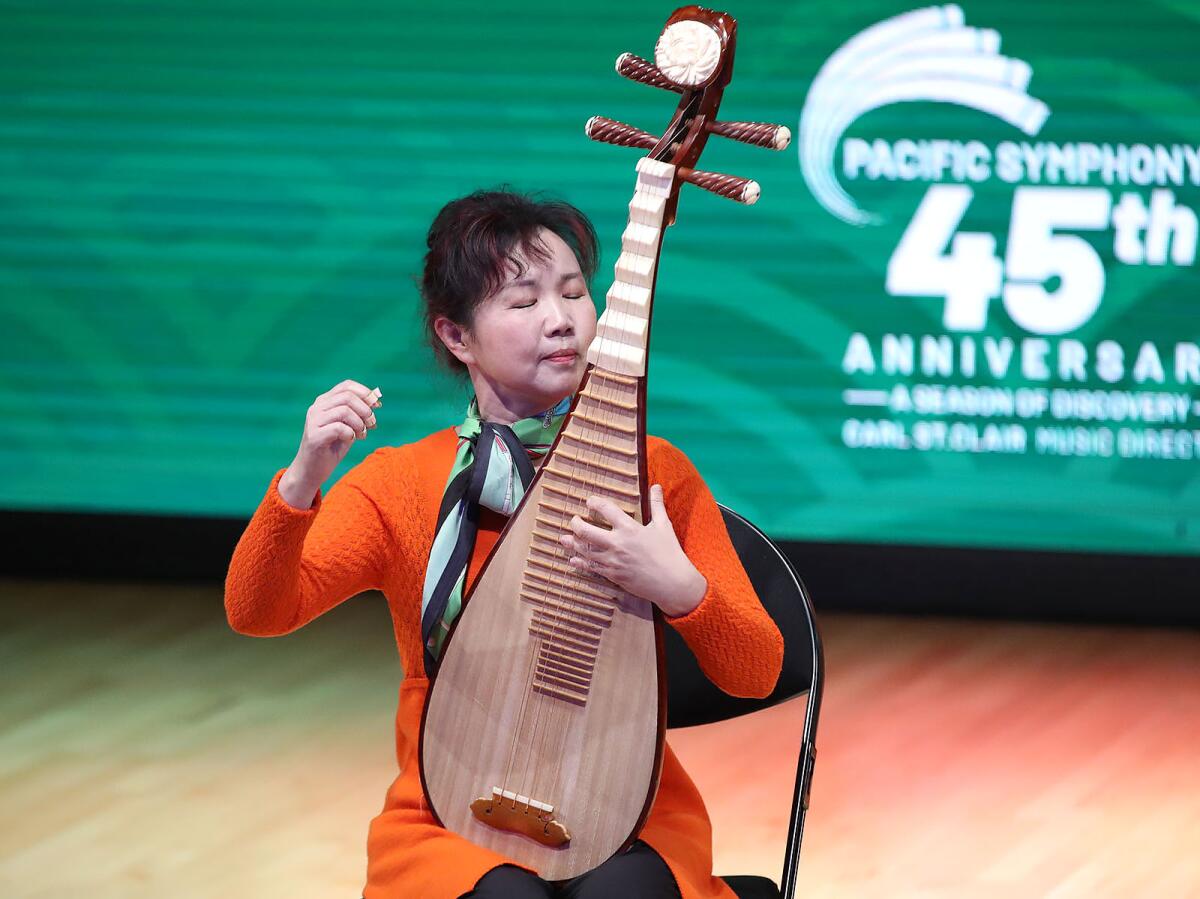The photograph features an Asian woman seated in a black folding chair, against a green backdrop that reads "Pacific Symphony 45th Anniversary, A Season of Discovery" in white writing. She appears to be in her 50s, her hair pulled back into a bun, and her eyes are closed. She is dressed in a bright orange long-sleeved top, possibly a tunic, and black pants. Draped around her neck is a scarf in shades of green and black.

The woman is playing a traditional Asian stringed instrument, possibly a pipa or a Japanese biwa, noted for its long neck and ornate carving at the top. This wooden instrument, which extends above her head, features an oval body and what appear to be four strings. She holds the instrument in her lap, with her left hand placed on the lower strings and her right hand poised to strum, capturing a moment of musical concentration. The setting resembles a basketball court due to the wood grain and coloring of the floor.